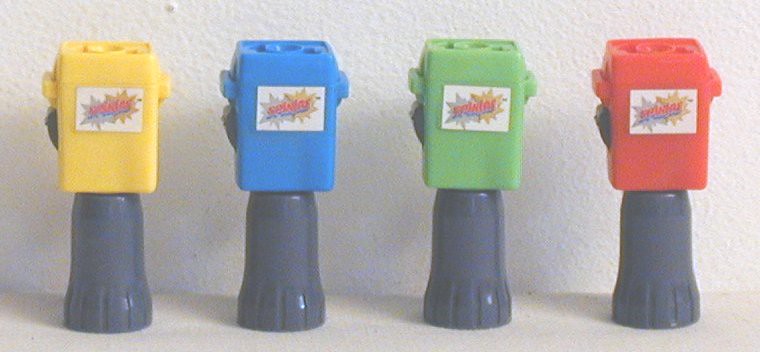In the up-close image, we see four small, colorful plastic objects that resemble toys. Each object is distinctly colored—yellow, blue, green, and red—and they are arranged from left to right. The tops of these 3D rectangle-shaped items, which look a bit like miniature garbage cans or cube-like structures, each have a hole on top and are adorned with white stickers. These stickers feature gray and yellow star patterns along with red and blue writing. Each toy has plastic handles on either side and they sit atop small gray cylindrical pedestals that widen at the base. The setting is a textured, bumpy white wall in the background, and the objects themselves are placed on a slightly darker, textured surface, likely a table or the ground.